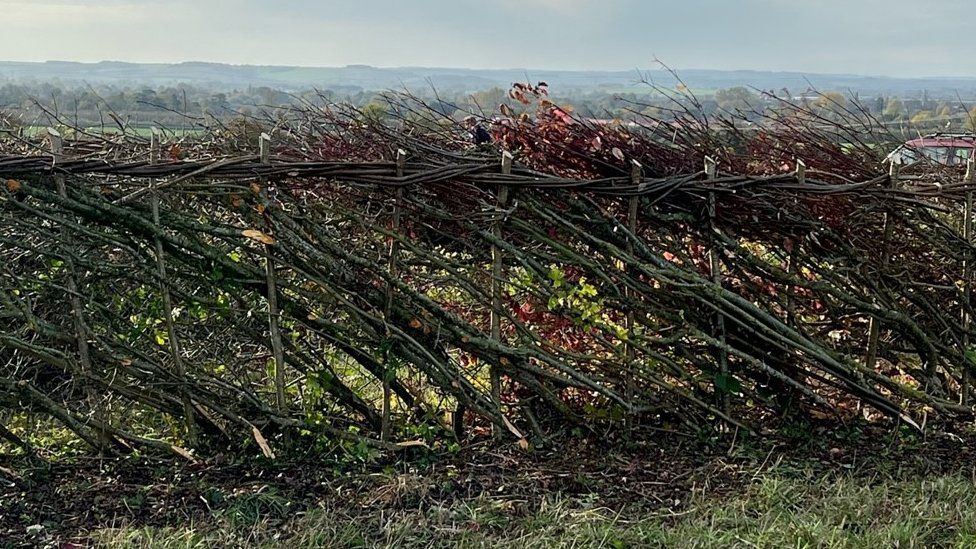The image captures a serene rural scene set in the countryside, likely farmland, with a prominent fence constructed from interwoven sticks, small branches, reeds, and foliage, creating a natural barrier and privacy screen. The fence dominates the foreground, extending across most of the photo, just above and beyond the sightline. In the distance, a picturesque landscape unfolds, featuring gentle hills and a dense forest under a somewhat dark sky that looms above what appears to be a level mountain range. At the bottom of the image, a lush grassy meadow spreads out, adding to the pastoral charm. Towards the middle of the photograph, a small figure, possibly a man, can be seen walking, though the details are minimal due to the size. To the right, just above the fence, the roof and parts of a red or maroon car peek into the frame, adding a subtle modern touch to the otherwise rustic setting. The natural elements entwining the fence include dark green, stick-like stems, possibly roots or fine vines, along with patches of red foliage, enhancing the texture and depth of this tranquil outdoor scene.